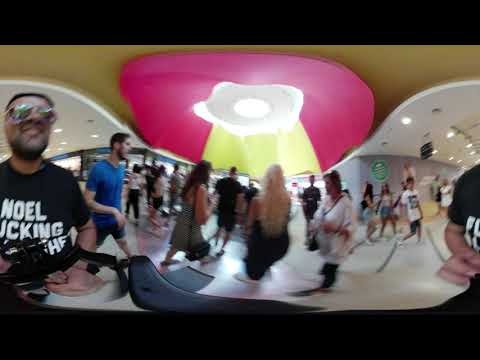In the bustling atmosphere of a large shopping center, a man captures a lively selfie using a selfie stick. He is wearing mirrored aviator sunglasses, a black shirt partially obstructed by the stick that bears the text "Noel Ucking HF," and has a short black beard and hair. The man is smiling brightly at the camera. The image reveals a vibrant crowd of people shopping and walking between stores. Prominently behind the man is another bearded gentleman in a blue t-shirt and gray shorts. A woman with blonde hair wearing a black dress has her head turned away from the camera. The ceiling, captivating with its yellow hue, showcases a central design resembling a pink, yellow, and white flower radiating with light. The frame of the picture exhibits black rectangles at the top and bottom, adding a distinct border to the busy and immersive scene. The atmosphere is so dynamic it almost feels like a 360-degree or virtual reality capture, enhancing the sensation of being amidst the throng. The bustling scene hints at a possible party or shopping extravaganza, enriching the photograph's lively essence.